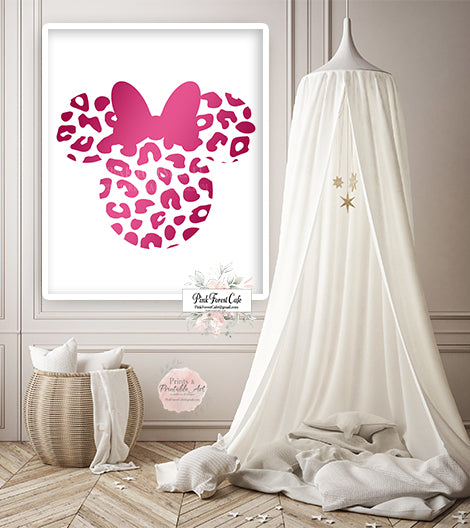The photograph showcases a charming room with a distinct Disney-themed decor. Central to the scene is a mini poster mounted on a white-paneled wall, featuring an outline of Minnie's head adorned with a leopard print in pink and white hues, and topped with a pink bow. The poster is framed in white and at the bottom bears the insignia "Pink Forest Cafe" accompanied by a logo. Adjacent to this is a suspended white canopy netting, which flows elegantly to the floor, creating a cozy reading nook cushioned with pillows and blankets, with a star mobile hanging in the center. The floor beneath features a beige or herringbone pattern. Additionally, positioned against the wall is a wicker basket containing pillows and a draped blanket or scarf, adding to the room's inviting ambiance.